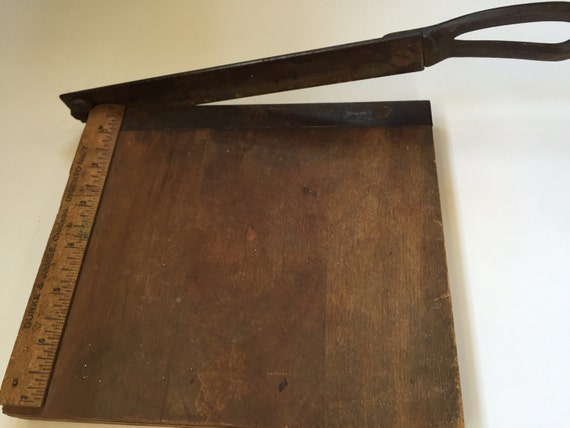This image depicts a vintage wooden paper cutter characterized by its square, light brown board showing notable wood grain, indicative of its aged and well-used condition. On the left side of the board, a lighter brown ruler extends from top to bottom, marked with black lines and numbers for precise measurements. The cutting blade, made of dark metal, is slightly raised at the top of the board and features an oval-shaped handle with a corresponding opening. This metal handle, designed for grip, integrates seamlessly with the flat edge of the blade. The background of the image contrasts between a white, cream-like hue with pronounced shadows to the right, and a light brown tint on the upper left, emphasizing the antique nature of the paper cutter.